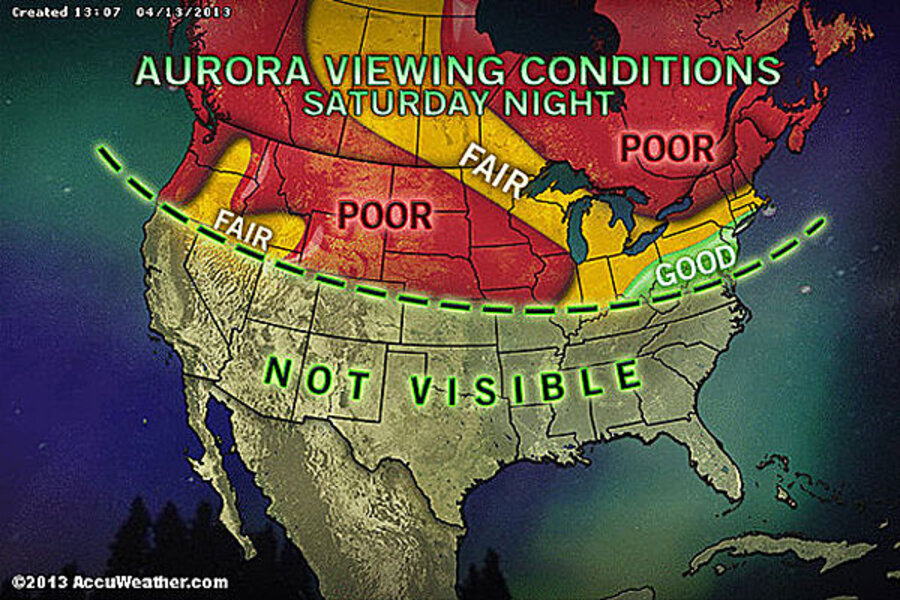The image is a detailed and colorful weather map displaying aurora viewing conditions for Saturday night. At the top of the map, it prominently features the title "Aurora Viewing Conditions" in green and white lettering, with "Saturday night" written underneath. The map itself covers the regions of Canada and the United States. In the northern parts of Canada and the United States, areas are highlighted in red, labeled as "poor" for aurora visibility. Moving slightly south, a larger swath stretching through parts of Canada and the northern United States, including the Great Lakes region, is shaded in yellow or gold, indicating "fair" visibility. A small area on the eastern side of the map is marked in green, representing "good" viewing conditions. An interrupted line runs across the map, demarcating these differently colored sections. The lower portion of the map, primarily covering most of the United States, is shaded in grey and labeled as "not visible," indicating no aurora visibility for these areas. Additionally, the map caption notes that it was created at 13:07 on 4-13-2013.